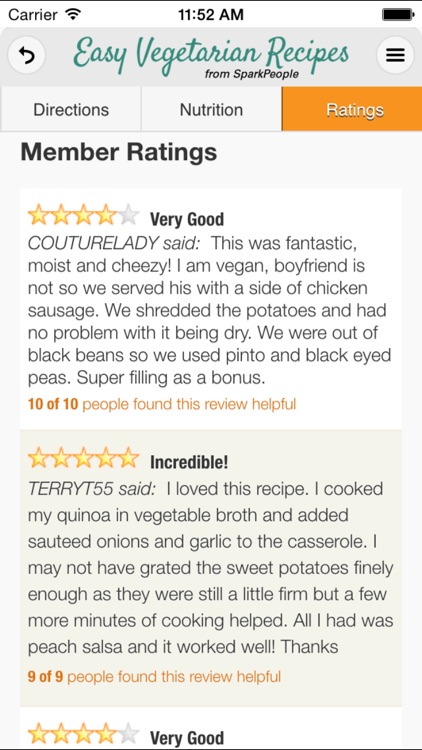**Caption:**

A screenshot from the "Easy Vegetarian Recipes" section on the Spark People website showcases member reviews for a featured recipe. The website's title, "Easy Vegetarian Recipes," is elegantly displayed in a green cursive font against a light gray background, with "From Spark People" written beneath in smaller, black text. In the upper right-hand corner, a menu icon is depicted as a white circle containing three black lines.

Below the title, navigation headings include "Directions," "Nutrition," and "Ratings," with the "Ratings" box highlighted in orange. The section prominently features member reviews. The first review, rated four out of five stars, is summarized as "Very good." User Couture Lady praised the recipe as "fantastic, moist, and cheesy," with the review noted as helpful by 10 out of 10 readers, indicated in orange text.

The subsequent review awards the recipe five gold stars, deeming it "Incredible." The final review, also rated four out of five gold stars, describes the recipe as "Very good."